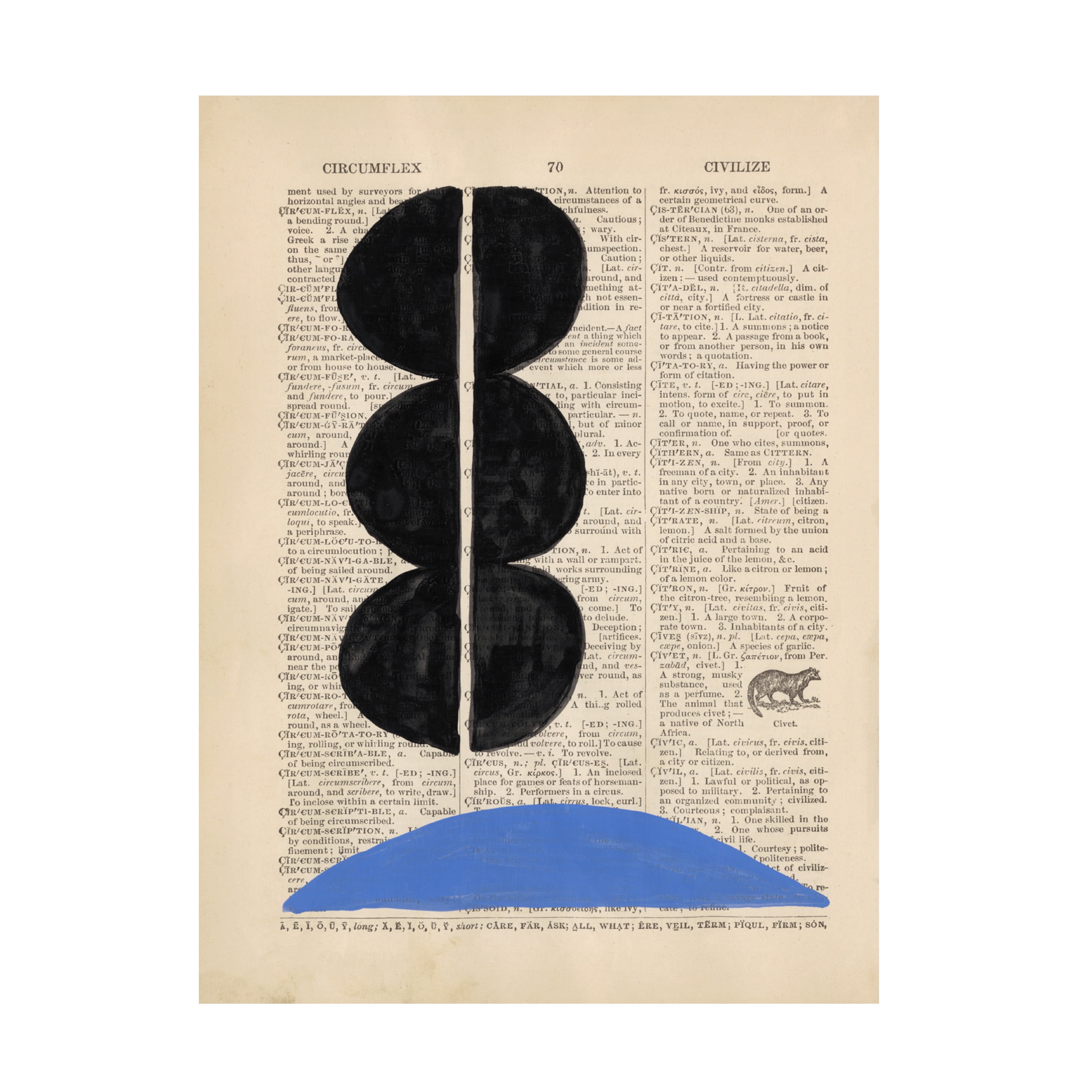The image is a mixed-media artwork featuring an old, yellowed dictionary page labeled as page 70. The page showcases definitions from "circumflex" to "civilize," organized in three columns filled with words starting with various CI- combinations and their definitions. Some words, including 'civilize,' are partially obscured. In the right column, there's an illustration of a civet accompanying one of the word definitions. The page is marked with three vertically aligned black semicircles near the top left, intersected by a blank vertical line, creating a pattern of incomplete circles. Below, at the bottom of the page, there's a large blue semicircle, mirroring the shape of the semicircles above. The paper itself seems worn, with evident stains and watermark, adding to the vintage aesthetic of the artwork.